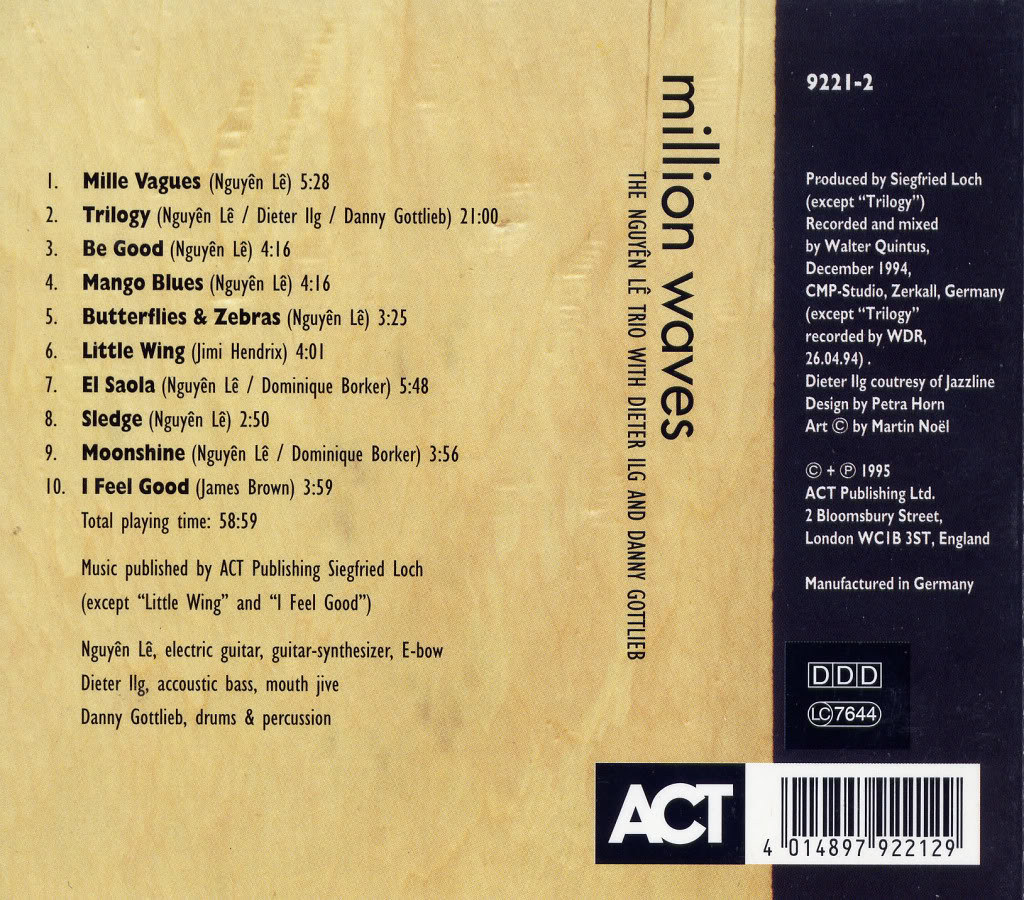This is the back cover of a musical recording CD or LP, divided into two sections. The left section, which occupies approximately two-thirds of the cover, has a beige background and lists the ten song tracks in order: Mie, Viggs, Trilogy, Be Good, Mango Blues, Butterflies and Zebras, Little Wing, El Saola, Sledge, Moonshine, and I Feel Good. Below the track list, there's a note that the music is published by ACT Publishing, Siegfried Locke, except for the tracks Little Wing and I Feel Good. It also specifies the band members and their instruments: the Nguyen Le Trio with Dieter Ilk and Danny Gottlieb.

The right section features a blue background that provides additional information about the CD. The text in this section is rotated 180 degrees and includes the title "Million Waves" and the artist lineup: The Nguyen Le Trio with Dieter Ilk and Danny Gottlieb. At the bottom right, spanning both the beige and blue sections, there is the ACT logo in black on a white box and a UPC code.